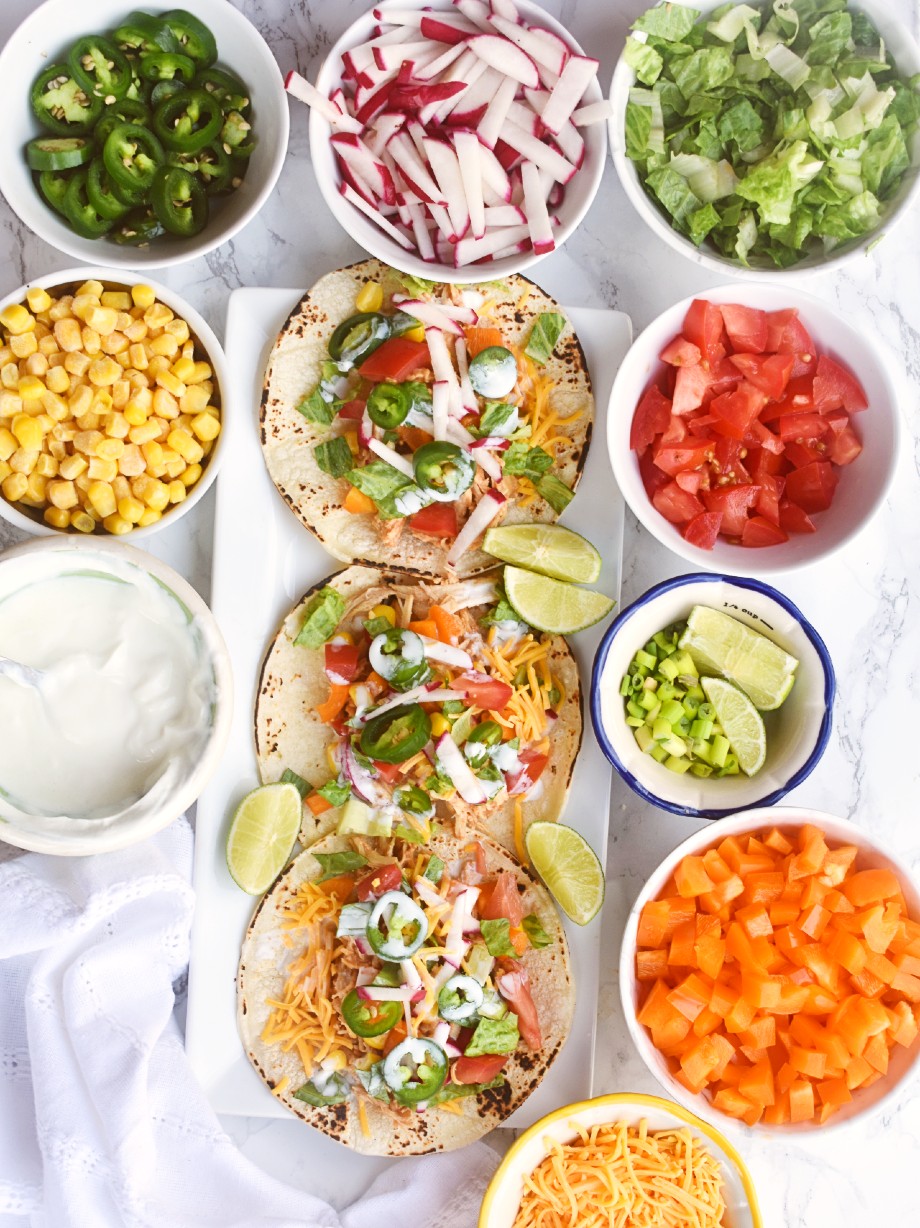The image is an overhead shot of a taco setup. In the center is a large white rectangular ceramic plate holding three open-face tacos on corn tortillas. Each taco is generously topped with a variety of ingredients including a cream sauce, sliced jalapenos, diced tomatoes, cilantro, shredded lettuce, and a mix of cheeses. Additional ingredients like sliced limes surround the tacos, enhancing their presentation. Around the plate, a number of bowls offer a selection of taco toppings, perfectly arranged for a DIY taco bar feel. These include sour cream, corn, diced radishes, more sliced jalapenos, shredded lettuce, tomatoes, scallions, chopped spring onions, slices of limes, orange bell peppers, and grated cheese. The setup rests on a large white piece of marble, with a semi-laced white tablecloth peeking in from the bottom of the image, giving it an elegant touch. No visible meat or protein can be clearly identified, suggesting a possible vegetarian theme or hidden layers of chicken underneath the vibrant toppings.